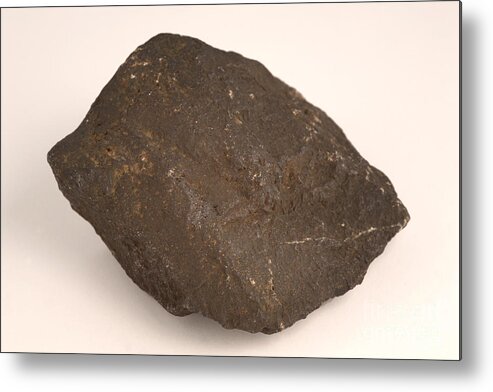The image portrays a large, rectangular rock set against a stark white background, devoid of any other elements. The rock exhibits a variety of earthy tones, predominantly shades of brown interspersed with black highlights and white flecks. The rock’s surface is characterized by numerous imperfections, including cracks on both the top and sides. A noticeable white vein, likely composed of a different mineral, runs through the rock, complemented by additional white and brown patches. The lower portion of the rock reveals a porous texture, suggesting the beginnings of fossilization, adding to its intriguing, rugged appearance.